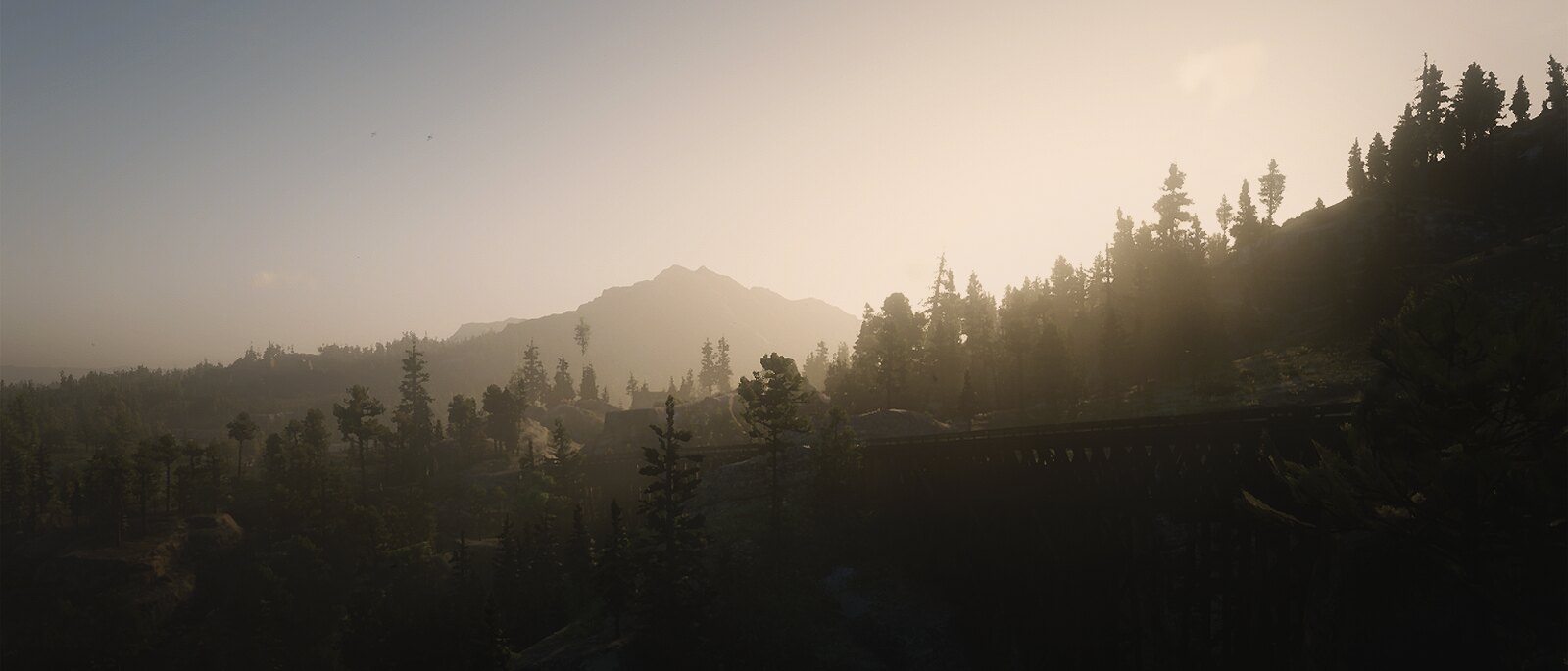A serene hand-drawn or painted image depicts a tranquil forest scene taken from a slight distance, capturing the early morning essence as the Sun begins to peek over a single mountain adorned with ridges. The forest, bathed in the soft pre-dawn light, reveals an enigmatic bridge, partly obscured by the semi-darkness, adding an element of intrigue. The dense forest stretches out in the background, creating a picturesque contrast against the silhouette of the solitary mountain. The overall atmosphere exudes a peaceful, almost ethereal quality, enhanced by the artist's skill in blending light and shadow.